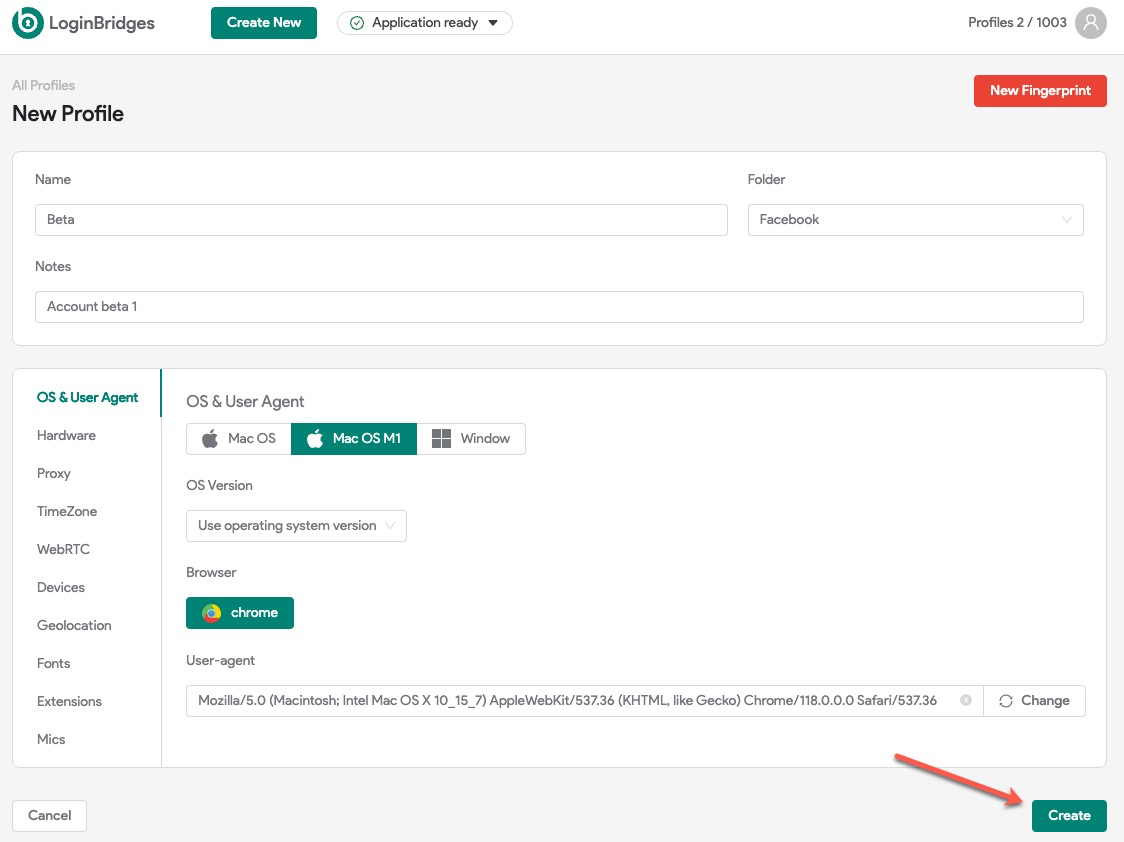This image is a detailed screenshot of the website or application called Login Bridges. The upper left-hand corner features a green circle with a "B" logo inside it, followed by the text "Login Bridges." Adjacent to this, a green button labeled "Create New" can be seen, as well as a green checkmark with the text "Application Ready" and a dropdown arrow beside it.

In the top right-hand corner, the text "Profiles 2 out of 1003" is displayed next to a grayed-out profile picture placeholder. Below this interface, the main content area of the website or application is visible.

In the upper left-hand corner of the main content area, tabs for "All Profiles" and "New Profile" are present. Correspondingly, in the upper right-hand corner, there is an orange button labeled "New Fingerprint."

The next section is divided into various input fields:
- The "Name" field currently contains the placeholder "Beta."
- The "Folder" field is labeled "Facebook."
- The "Notes" field contains the text "Account Beta 1."

Below these input fields, there is a menu of clickable sections, with the "OS and User Agent" section currently highlighted in green, while the others are grayed out. The grayed-out sections include Hardware, Proxy, Timezone, WebRTC, Devices, Geolocation, Fonts, Extensions, and Mics.

In the highlighted "OS and User Agent" section, the details include:
- "Mac OS M1" as the operating system
- "Use Operating System Version" as an option
- "Browser" set to Chrome
- "User Agent" details.

Finally, in the bottom right-hand corner of the screen, there is a reddish-orange button labeled "Create" with an arrow pointing downward towards it.